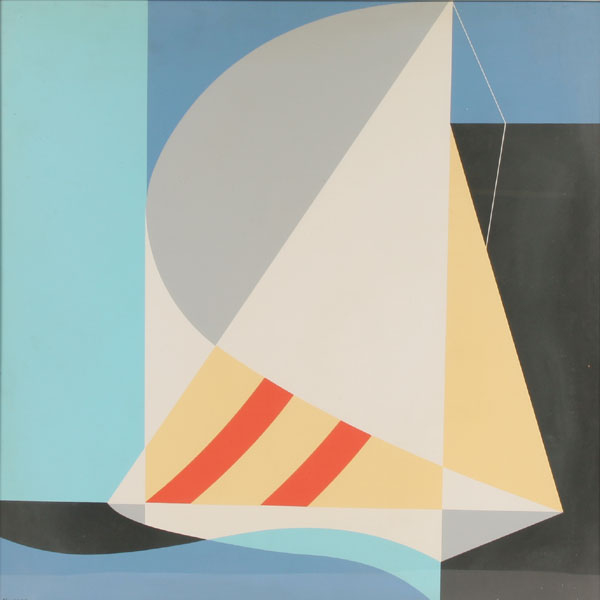This image is an abstract mixed media piece that creates the illusion of a sailboat on the water. Central to the image is a large white triangle with a beige base and two red stripes, symbolizing the sail, set against a blue background. To the left of this triangle is a significant oval half-circle shape in gray. The right side is juxtaposed with another yellow triangle against a black backdrop, contributing to the sailboat imagery. A sizable strip of blue occupies the left-hand side, enhancing the water illusion. The bottom features a wavy blue curve above a black and white strip, further fortifying the sense of waves. The overall color palette is neutral and muted, including hues of teal, blue, light blue, dark blue, gray, soft gold, and orange. Surrounding the central sailboat structure are various other symmetrical shapes, such as triangles, circles, and rectangles, arranged harmoniously on the multicolored canvas. Although geometrical and structural, the dynamic curves and placement of shapes suggest movement through water, making the abstract illustration evocative and engaging.